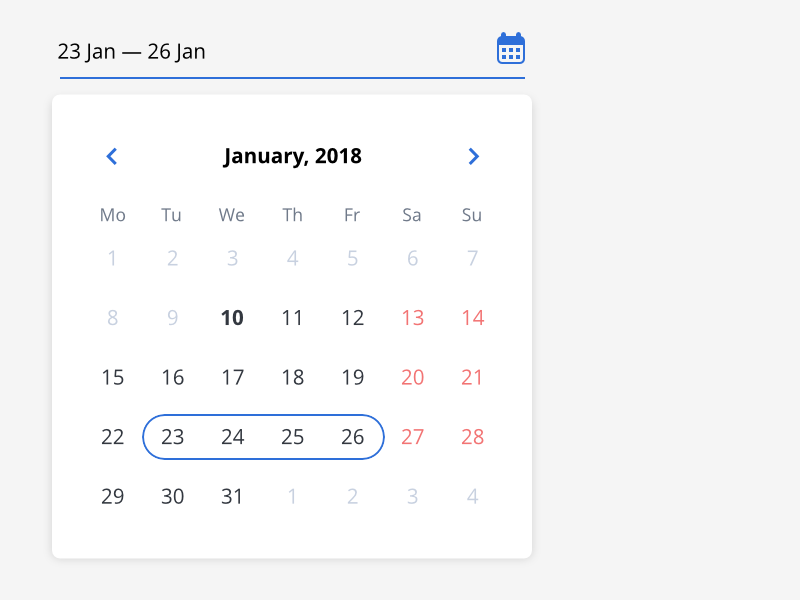The image appears to be a screenshot from a digital calendar application, displaying the month of January 2018. The calendar is set within a light gray, slightly raised rectangular interface. At the top of the white calendar box, centrally aligned, it reads "January 2018," with navigation arrows on the left and right sides for changing the month.

The days of the month are displayed in a grid format. The dates from January 1st to January 9th are shown in a light gray font, indicating they are from the previous month. January 10th is highlighted in bold black, while January 11th and 12th are in a lighter black font. January 13th, 14th, 20th, 21st, 27th, and 28th are marked in red, suggesting these could be weekends. The dates from January 15th to January 19th and January 22nd to January 26th are in a standard black font. The period from January 23rd to January 26th has been circled in blue, indicating a specific focus or event spanning these dates.

Above the calendar, in the upper left corner of the interface, it prominently notes "January 23rd to January 26th," highlighting the key period of interest. This suggests that the user has specifically selected or marked these dates for attention.